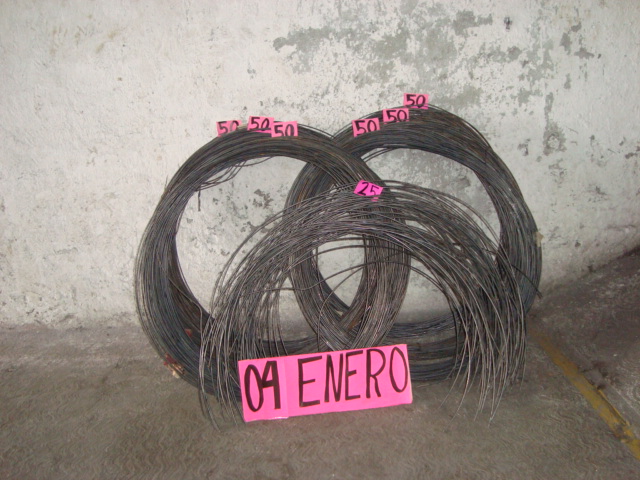The color photograph appears to be taken in a garage or basement, featuring a weathered, peeling concrete wall and a dirty concrete floor marked with footprints and squiggly lines. Leaning against the concrete wall are three bundles of wire. Two of these bundles are full circles, each with hot pink post-it notes marked "50-50-50." The third bundle is a semi-circle with a hot pink post-it note that says "25." In front of the wire bundles is another note that reads "04 enero" (Spanish for January 4th), written in black marker. The scene suggests an organized, yet casual storage or sale setup, possibly for a construction or building project, indicated by the specific lengths and quantities noted on the post-its.